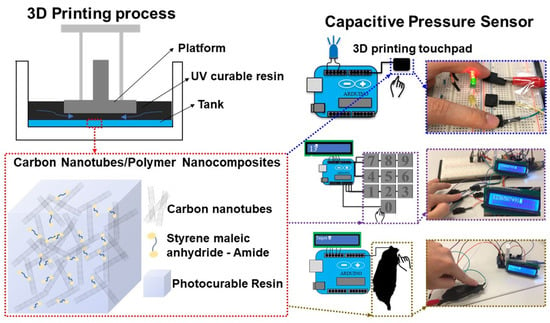The image is a detailed color technical diagram illustrating the 3D printing process and its components. In the upper left corner, the text reads "3D printing process," setting the context for the intricate visual below. At the center of the diagram, a white, black, blue, and gray schematic depicts a box-like apparatus with an upside-down T shape labeled as "platform." Above this is a frame structure, while below it sits a black section indicating "UV curable resin," and beneath that, a blue line marked "tank."

Adjacent to this central component is a red-dotted box titled "carbon nanotubes/polymer nanocomposites," containing a white cube with gray zigzags and dark gray and yellow spots. This cube is further explained with labels including "carbon nanotubes," "styrene maleic anhydride amide," and "photo curable resin."

On the left-hand side, the diagram is titled "capacitive pressure sensor" and features a series of blue, gray, and green diagrams. Complementing these diagrams are three photographs aligned vertically on the right. The top photograph shows a Caucasian hand holding two black objects connected by wires. The second image features fingers managing an array of wires, black connectors, and two illuminated blue screens. The third photo depicts the hand pressing a black node linked by multicolored wires to another blue screen and additional components. This arrangement provides a comprehensive visual guide to the 3D printing process, from the technical setup to the intricate details of the printed materials and sensors.